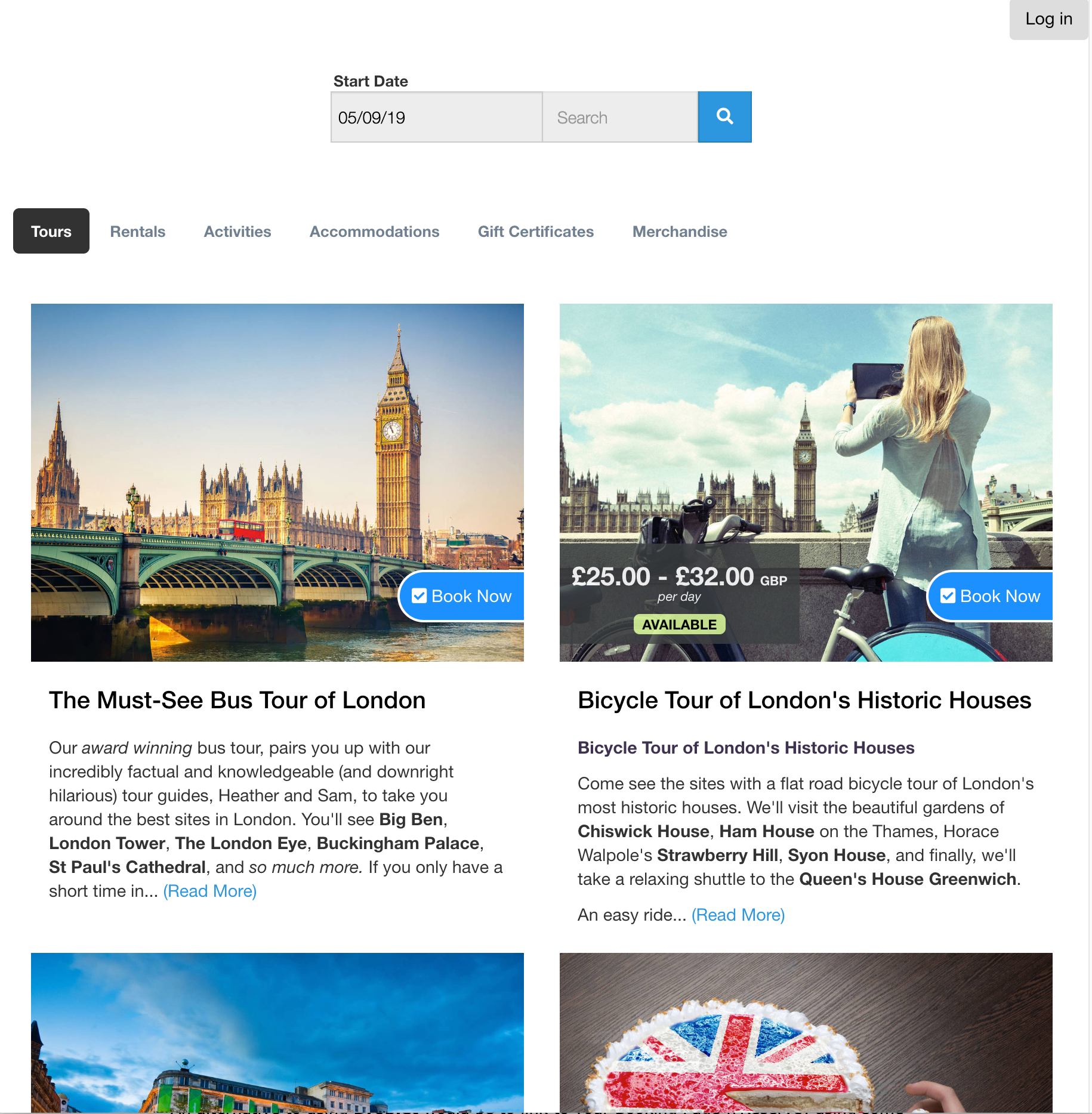This is a detailed screenshot depicting a user interface for booking tours and activities. 

At the top right corner, there is a gray "Log In" button. Below in the center, the screen prominently displays a "Start Date" section with a gray rectangular box filled with the date "05/09/19". Adjacent to this box is another gray box labeled "Search", accompanied by a small blue box with a magnifying glass icon indicating search functionality.

Further down, there are several categories available for selection: Tours, Rentals, Activities, Accommodations, Gift Certificates, and Merchandise. The "Tours" category is currently highlighted with a black background box.

Beneath these categories, two large images are displayed. The first image showcases the iconic Tower of London, titled "The Must-See Bus Tour of London". The description beneath highlights an award-winning bus tour featuring humorous and knowledgeable guides named Heather and Sam. Key landmarks mentioned include Big Ben, Tower of London, the London Eye, Buckingham Palace, and St. Paul's Cathedral. The description ends with an invitation to "read more" in blue text.

The second image features a girl taking a picture with her tablet, with the Tower of London in the background. She has blonde hair, wears a light blue shirt and blue jeans, and is accompanied by a bicycle with blue spokes. The tour, priced between £25 to £32 per day, offers a "Bicycle Tour of London: London's Historic Houses," mentioning sites like Strawberry Hill and Queen's House in Greenwich. Both images include a "Book Now" button.

Additionally, the preview of two more images is partially visible at the bottom. The left image hints at a building against a beautiful blue sky, while the right image seems to feature a circular cake adorned with the British flag design.